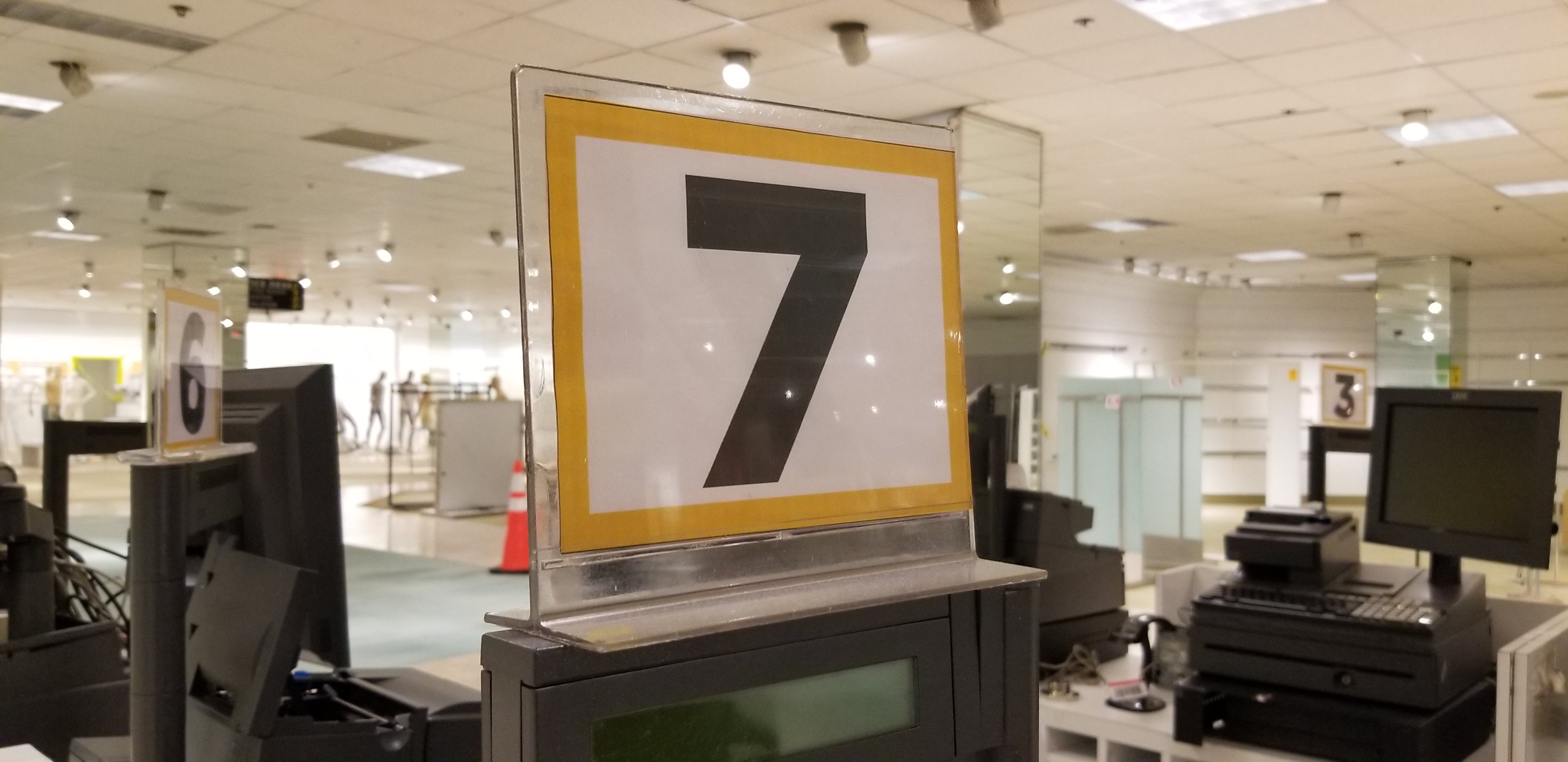The image appears to be taken inside an electronics store, featuring a variety of devices such as computers, laptops, and possibly stereos. The ceiling is made of white panels with built-in lights, along with several additional lights protruding from it. Various walls within the store display large numbered signs, each outlined in yellow and white, with bold black digits. A prominently visible sign at the front showcases a '7', while another similar sign with a '6' can be seen from different angles. Additionally, a sign with a big '3' is located towards the back. Mannequins are placed further into the store, and to the left, there is a screen—potentially a computer monitor or TV. A collection of cords is also visible. In the center of the store, mirrored partitions create a reflective effect, adding to the intricate layout of the space.